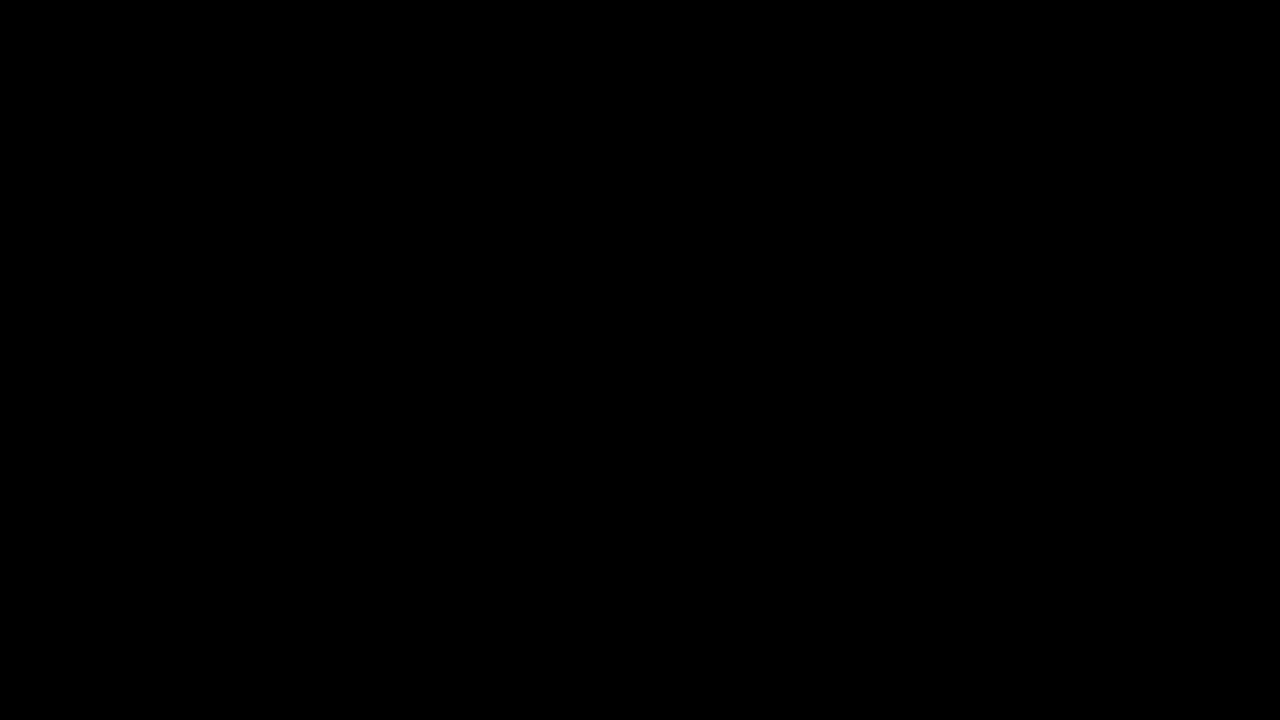This image is a completely black rectangle with no discernible objects, colors, or text anywhere. The black color fills the entire space from edge to edge, creating an uninterrupted void. The matte finish of the black adds to the sense of emptiness and starkness, with no reflections or specks to break the uniformity. Its aspect ratio shows that it is longer from side to side than it is from top to bottom. The uninterrupted black space produces an eerie sensation of emptiness or loss, almost as if staring into a void or an abyss. In the context of a computer screen, the contrast between the black image and the white background makes it appear even more like a void you could fall into, enhancing the unsettling feeling of boundless emptiness.